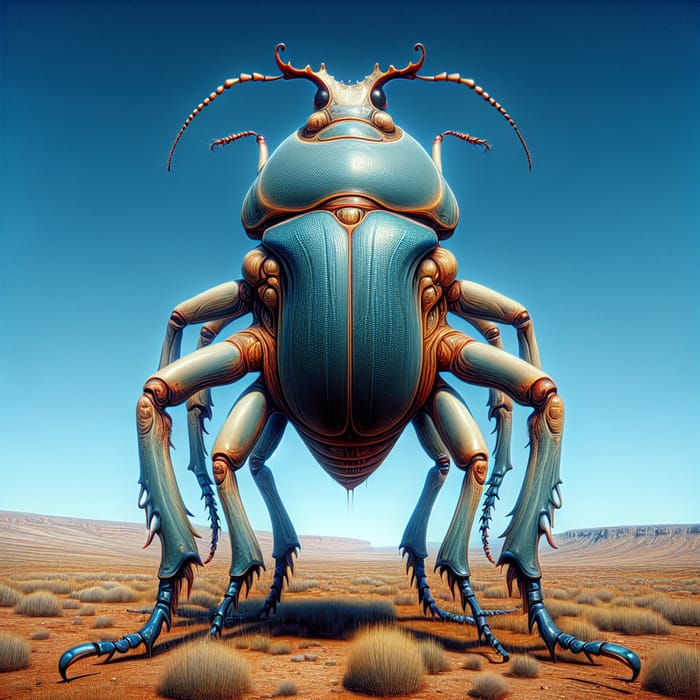This digital artwork showcases a prominent giant bug positioned at the center of the image, standing on a mostly flat and sandy desert terrain dotted with small plants, such as weeds or shrubs. The creature, resembling a beetle or ant-like organism, features a unique body structure with eight legs—an unconventional deviation from the traditional six. It is primarily light blue with distinct red markings around the connective tissues and knee areas on its legs. The bug's body is predominantly tall rather than long from this perspective, and it stares directly ahead with two prominent black eyes. Additional details include short appendage-like structures below the eyes and long whisker-like appendages above its head. The backdrop contrasts vividly with the bug, presenting a clear blue sky with subtle gradients of light and dark blue hues, and distant hills or mountains accentuating the horizon.